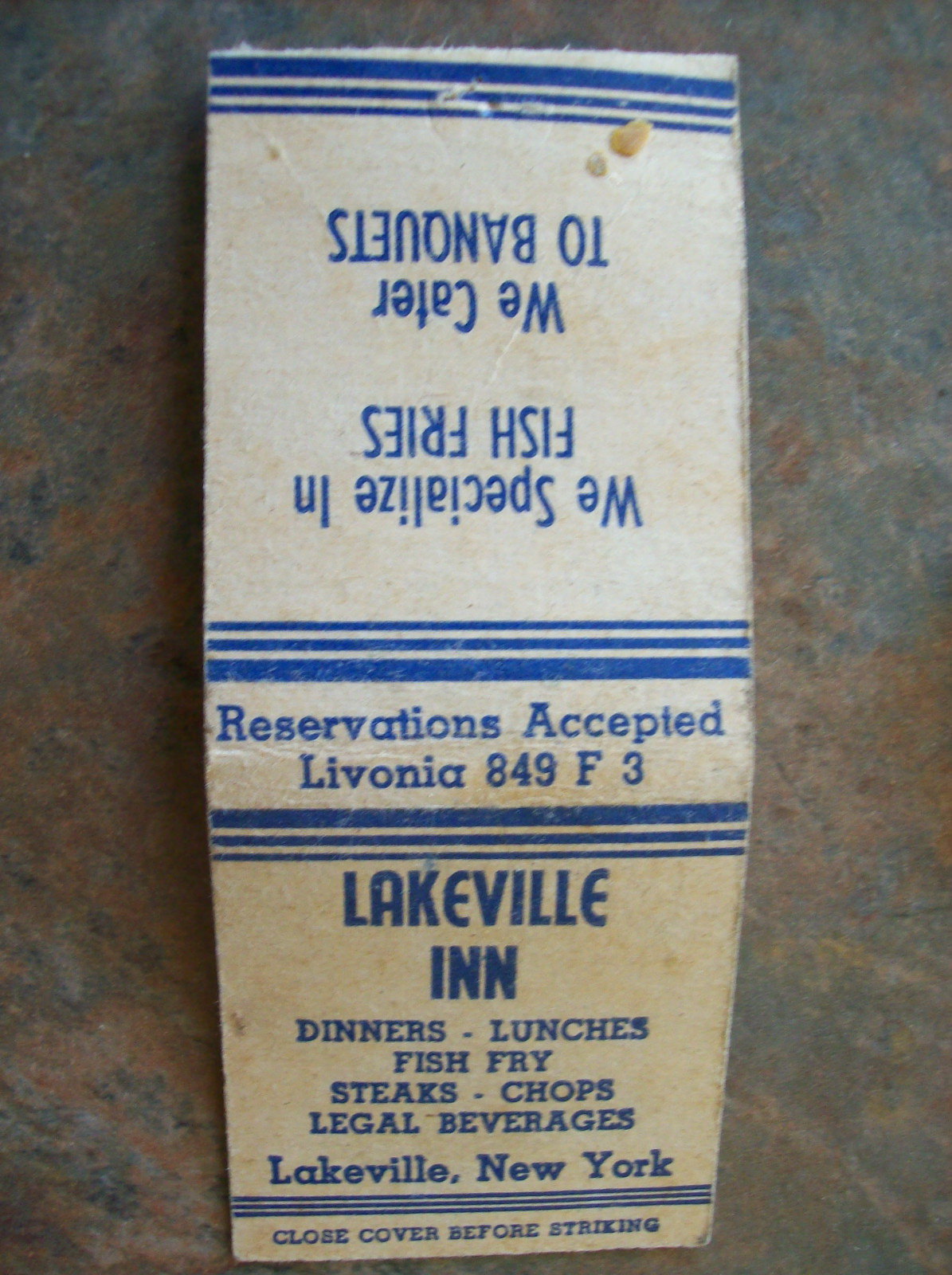The image shows an aged, white matchbook laid open on a dark granite or marbled surface, creating a stark contrast with varying shades of blue and brown in the background. The matchbook's front and back cover are both visible, adorned with notable wrinkles along the middle. The cover, having yellowed with time, displays blue text and stripes on both the top and bottom sections. Clear text reads: "Reservations Accepted, Livonia 849F3. Lakeville Inn. Dinners, lunches, fish fries, steaks, chops, legal beverages, Lakeville, New York." Additional upside-down text at the top states: "We specialize in fish fries. We cater to banquets." The classic matchbook reminder, "Close cover before striking," is also clearly seen.